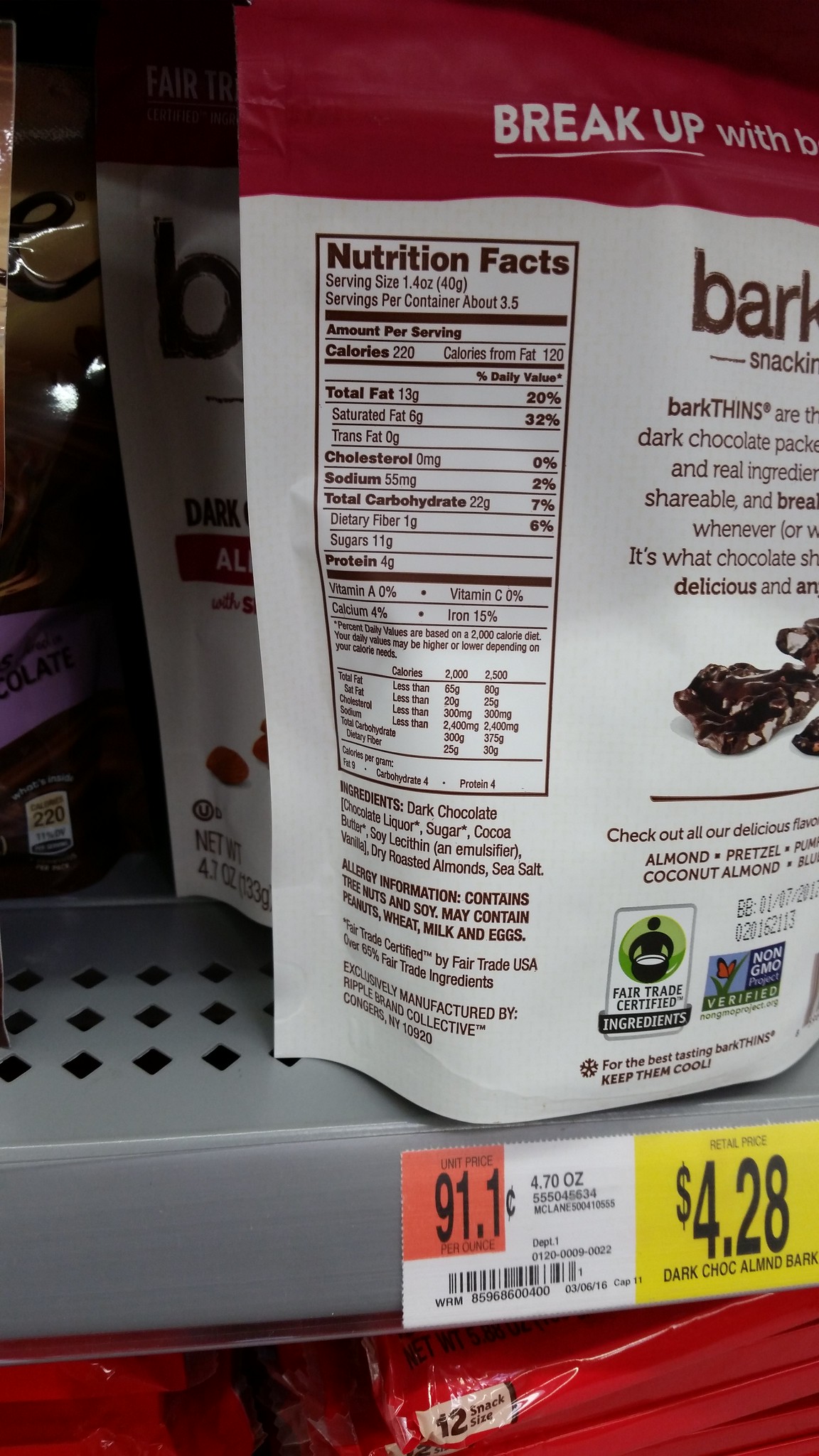The image depicts a gray-colored shelf displaying various products. A red package at the bottom stands out, labeled "12 Snack Size." The focal point, however, is on the back of a package of dark chocolate almond bark positioned above it. 

The almond bark packaging features a dual-colored design with a red border across the top and a predominantly white body accentuated by brown text. A fragment of the packaging’s tagline, "Break up with B," is visible before being cut off in the image. Detailed nutritional information is prominently displayed: serving size is 1.4 ounces with approximately 3.5 servings per container. Each serving contains 220 calories, with 120 calories from fat. Key nutritional content includes 13 grams of total fat (6 grams of which are saturated), zero trans fat, zero cholesterol, 55 milligrams of sodium, 22 grams of carbohydrates, 1 gram of dietary fiber, 11 grams of sugar, and 4 grams of protein. Additionally, the package specifies the presence of 4% calcium and 15% iron, with no Vitamin A or C content.

The ingredients are listed as dark chocolate, chocolate liqueur, sugar, cocoa butter, soy lecithin, dry roasted almonds, and sea salt. An allergen warning indicates that the product contains tree nuts and soy, and may also contain traces of peanuts, wheat, milk, and eggs. The price tag affixed to the yellow label below the package reads $4.28.